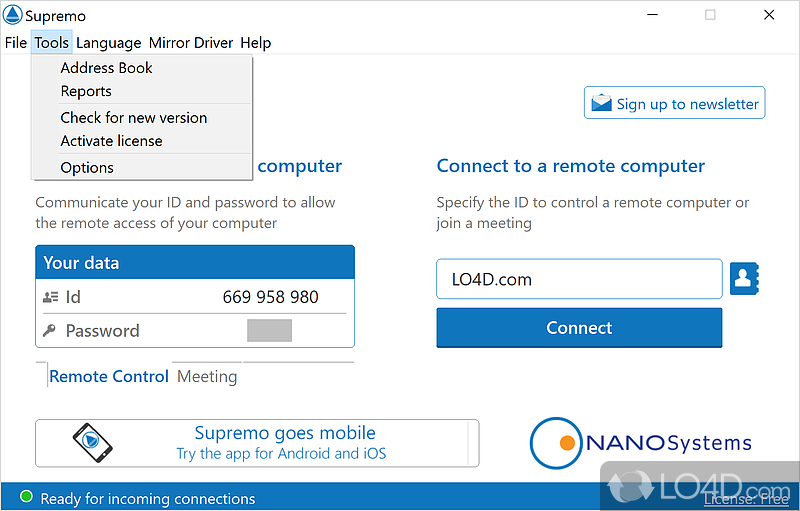This screenshot depicts a user interface with a clean, white background outlined in light gray, designed in a rectangular shape that is longer horizontally. In the upper left corner, there is a logo consisting of a blue circle enclosing a blue triangle, accompanied by the black text "SUPREMO." 

Below the logo, there is a horizontal menu bar listing the following options from left to right: "FOOL," "FILE," and "TOOLS." The "TOOLS" option has a dropdown menu that lists additional items: "ADDRESS BOOK," "REPORTS," "CHECK FOR NEW VERSION," "ACTIVATE LICENSE," and "OPTIONS."

Continuing to the right of the "TOOLS" menu, there are further options labeled "LANGUAGE," "MIRROR," "DRIVER," and "HELP."

In the lower right corner of the screenshot, there is a blue circle enclosing a small yellow circle. To the right of this icon, the text "NANO SYSTEMS" is displayed in blue. Beneath this, the text "4D.COM" and "LICENSE. FREE" are also visible.

At the bottom left corner, there is a blue footer displaying the message "READY FOR INCOMING CONNECTIONS," with a small green circle to the left of this text. Above this footer, within a white box, a promotional message reads, "SUPREMO GOES MOBILE. Try the app for Android and iOS."